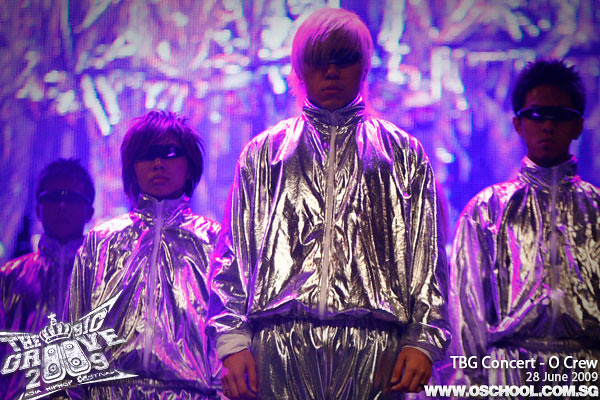The image is a rectangular advertisement for "The Big Groove 2009" concert featuring four individuals standing in a V formation. Each person is dressed in a full-body silver lamé jumpsuit with a front zipper and dark sunglasses, exhibiting a poker-faced expression. The band members have unique and flamboyant hairstyles: one with pink hair, another with spiky dark hair, the third with purple hair, and the last with short dark hair. The background is illuminated with blue and pink lighting, contributing to a shiny, electrifying atmosphere. In the top left corner, the logo for "The Big Groove 2009" with a small crown is prominent. The bottom right corner contains the text "TBG Concert-O Crew, 28 June 2009, www.oschool.com.sg" in white. The figures' heads are inclined at different angles, suggesting a dynamic pose, and they are potentially a Singaporean boy band.